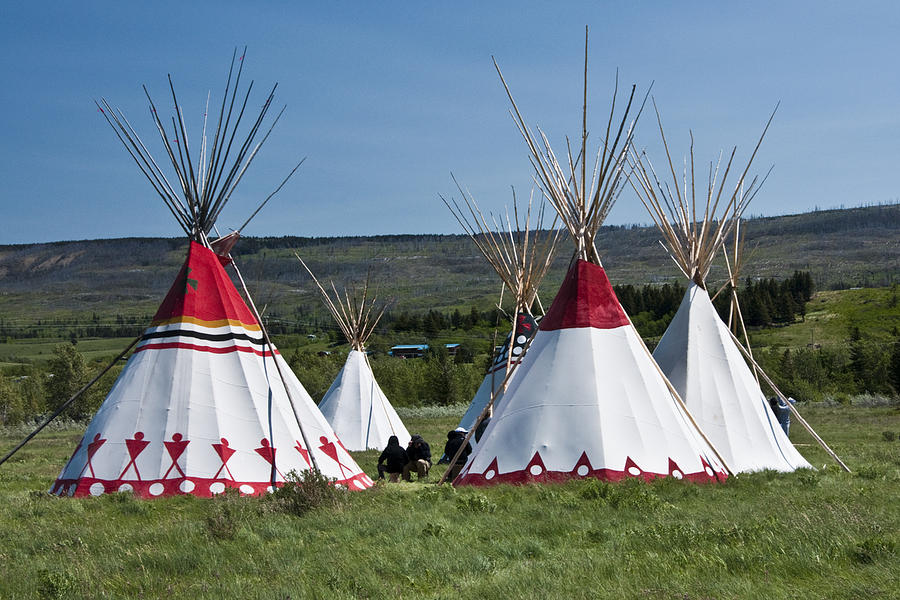The photograph showcases a serene scene of five teepees arranged in a green, unmowed field. The grass is dotted with weeds, and the backdrop features gentle hills with scattered evergreen trees under a clear blue sky. The teepees, predominantly white, display distinctive designs: the leftmost one is adorned with a red tip, orange, white, black, and red stripes, along with simplified depictions of people around its base. The rightmost teepee has a cherry-toned red tip, a red bar at the bottom with equidistant triangles containing white circles. The central teepee is plain white. In the space between the first pair of teepees, three indistinguishable shadowy figures kneel. The remaining teepees, partially obscured, include one plain white and another with a black tip featuring a red cross and white circles. Wooden poles extend from the tops of each cone-shaped teepee. The overall arrangement and design elements suggest a blend of traditional craftsmanship and modern influences.